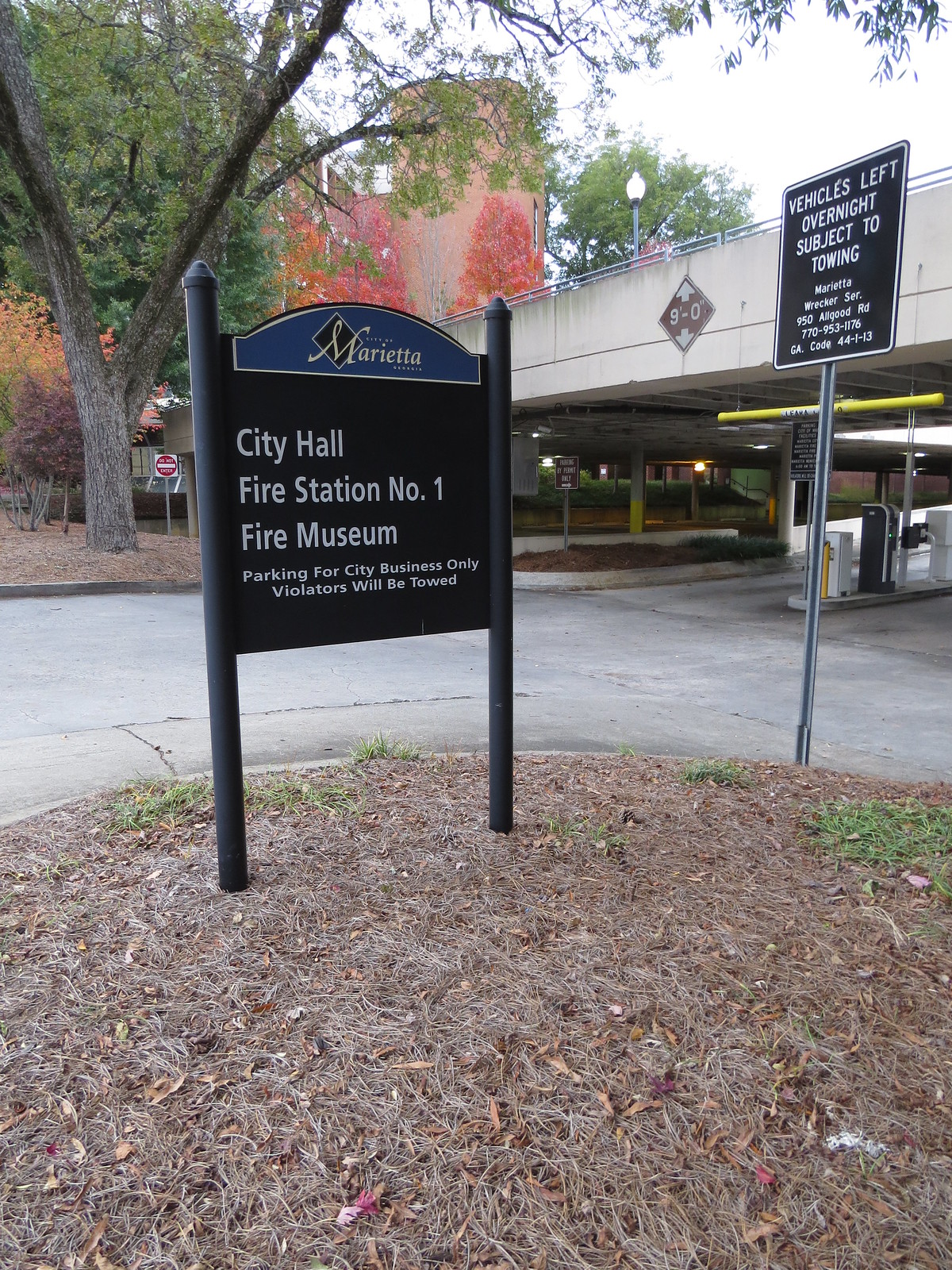In this detailed outdoor daytime photograph, the setting is in front of what appears to be a multi-story parking garage. In the foreground, prominently displayed on a patch of dead grass, is a sign with cursive writing at the top that reads "Marietta City Hall." Below it, in block letters, it designates "Fire Station Number 1 Fire Museum," followed by a cautionary note: "Parking for city business only. Violators will be towed."

To the right of this main sign, another black sign stands, warning, "Vehicles left overnight subject to towing," with additional details including a partial address, "Marietta Wrecker Service, Allgood Road," a phone number, "770-953-1176," and "GA Code 44-1-13."

A diamond-shaped, yellow traffic sign is mounted on a walkway above the parking garage, indicating a clearance height of "9'0"." The background reveals some trees, mostly green with a scattering of orange foliage, hinting at the onset of autumn. The multi-story building behind the trees is light brown under a gray, overcast sky, completing the scene.